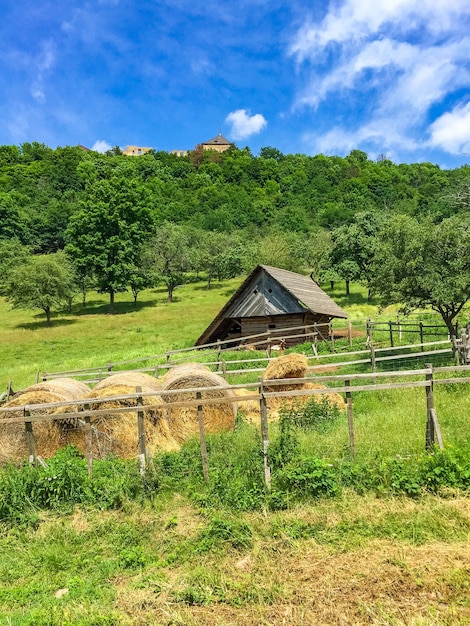On a partly cloudy day, this photograph captures a serene farmland landscape. In the foreground, thin wooden fencing encloses several yellow and tan rolled bales of hay, sitting at the base of the fence. Adjacent to this area, another fenced-in section lies empty, while further back stands a small, gray triangular shed with a uniquely slanted roof that slopes all the way to the ground on the left side. The grassy terrain is a mix of bright green with patches of tan, extending towards the background. Beyond the shed, an uphill slope leads to a densely packed tree line, and two additional tan structures can be seen peeking above the lush greenery. The sky is a beautiful blue adorned with scattered white clouds that are more concentrated on the right side of the image, enhancing the idyllic countryside setting.